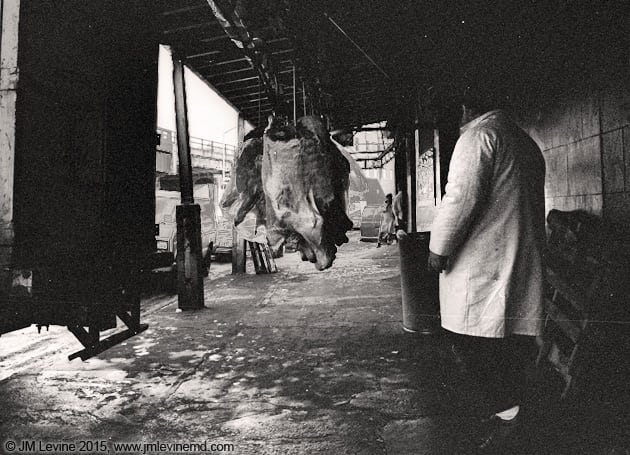In this black-and-white photograph, a heavyset man in a light-colored trench coat and dark boots, with a piece of his white socks visible, is walking towards several large slabs of meat hanging from hooks under an overhanging roof. The setting appears to be outside, possibly a meatpacking district or a slaughterhouse, with a street and parked cars on the left-hand side and an elevated railroad visible in the background. The area is dimly lit despite the daylight outside, suggesting strong contrast in the photograph's exposure. To the right, there's a building with some pallets against its wall. Another person can be seen further down the sidewalk, near what looks like a dumpster. The ground outside appears to be cold, possibly covered with snow or ice.